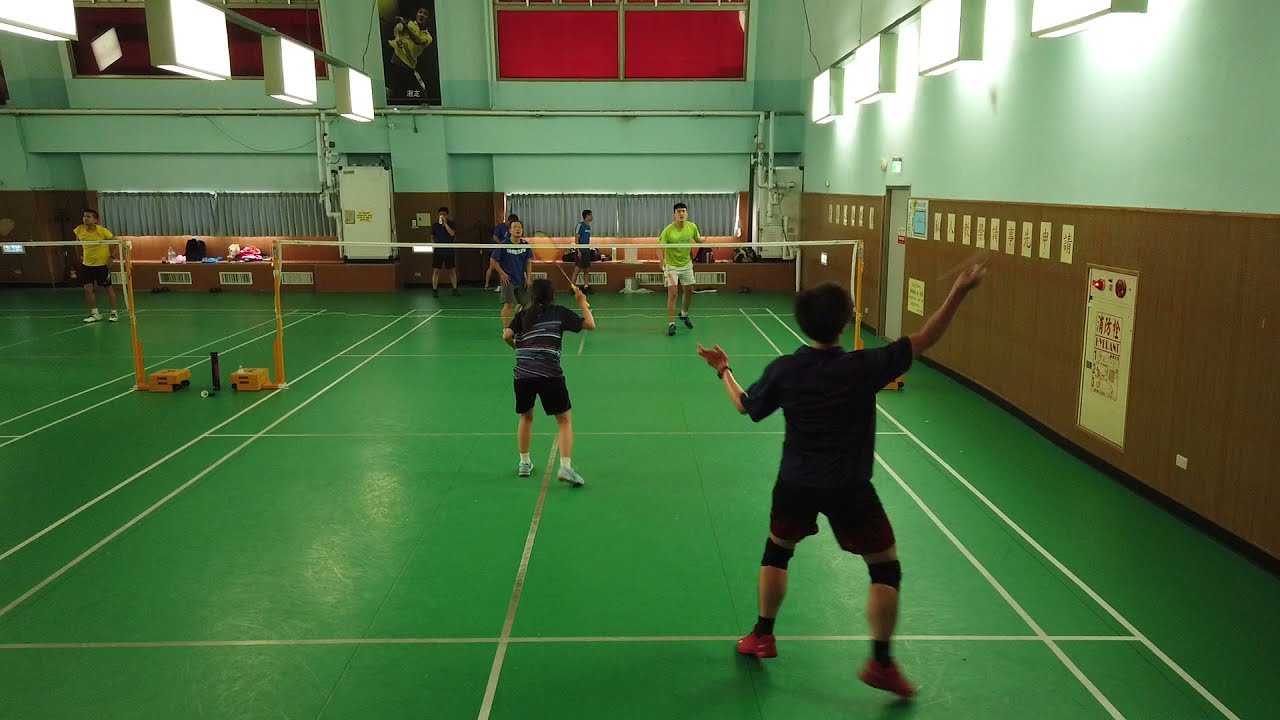This photograph captures an indoor badminton court situated in a gymnasium. The floor of the court is painted bright green with white boundary lines, and a white net with orange supports divides the court. There are four players actively engaged in a match: two on each side of the net. On the closer side to the viewer, the player in the foreground, dressed in black shorts, a black top, and red shoes, appears to be striking the shuttlecock, while his partner, also clad in dark clothing with white shoes, is positioned slightly to his left. Their opponents on the far side consist of one player in white shorts and a green shirt and another in dark attire.

Positioned vertically in the composition, the court is flanked by walls that exhibit a range of colors including red, light green, and light brown. The walls also feature attached lights that illuminate the playing area. Above the court, near the ceiling, there are visible red-colored windows. Additional elements in the background include three more people who seem to be casually moving around or observing the game. On the left edge of the image, a portion of another badminton court can be seen, suggesting that this might be a training facility. The dynamic movement of the players and the vibrant colors highlighted in the image give a sense of recreational activity and energy.